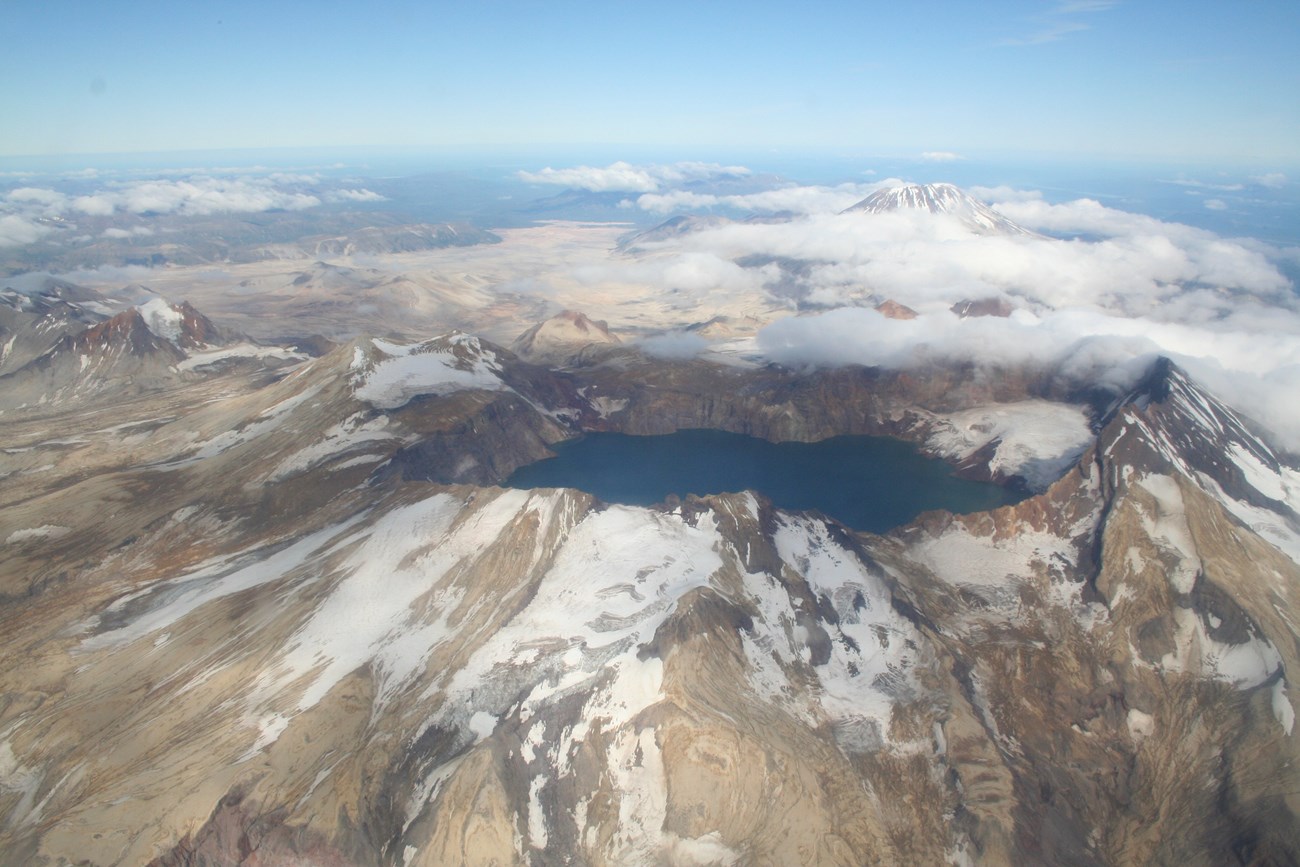This aerial photograph, likely captured from a plane, helicopter, or drone, offers a breathtaking view of a mountaintop crater with a sizeable pool of water nestled within. The peak is dusted with a light layer of snow that adds a delicate contrast to the predominant yellows, beiges, and occasional grays of the rugged mountain landscape. In the distance, a few taller mountain peaks can be seen piercing through the cloud cover. Despite being one of the largest craters and bodies of water in the image, the setting exudes a majestic serenity, emphasized by the snow's subtle presence that highlights the contours of the mountaintop.